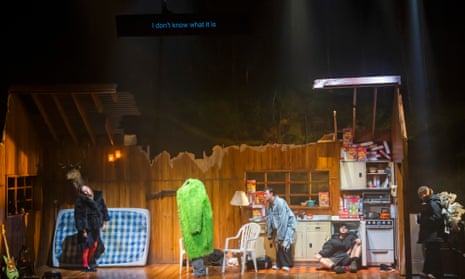The image captures a small, dimly lit theater set designed to resemble a dilapidated kitchen from a bygone era, perhaps evoking a sense of poverty or hardship reminiscent of 1930s Appalachia. The setting appears torn or damaged, with a dark blue and light blue checkered mattress leaned against a wooden wall on the left, next to a green guitar. 

Central to the scene is an enigmatic figure wearing a green, furry coat that obscures their head, giving them a headless appearance reminiscent of a character from a whimsical play. Nearby, an individual dressed in a black fur garment and red hose stands in front of the mattress, while another person hunched over in a jean jacket is positioned in the middle. 

On the right side, a person in a blue shirt and dark pants stands near a stove and cupboards, with some food items visible, including cereal boxes in a pantry. There are two white chairs in the middle of the floor, and another person can be seen sitting beside the stove and within one of the cupboards. The scene exhibits a mix of typical household items and peculiar behavior, contributing to its theatrical and somewhat surreal atmosphere.